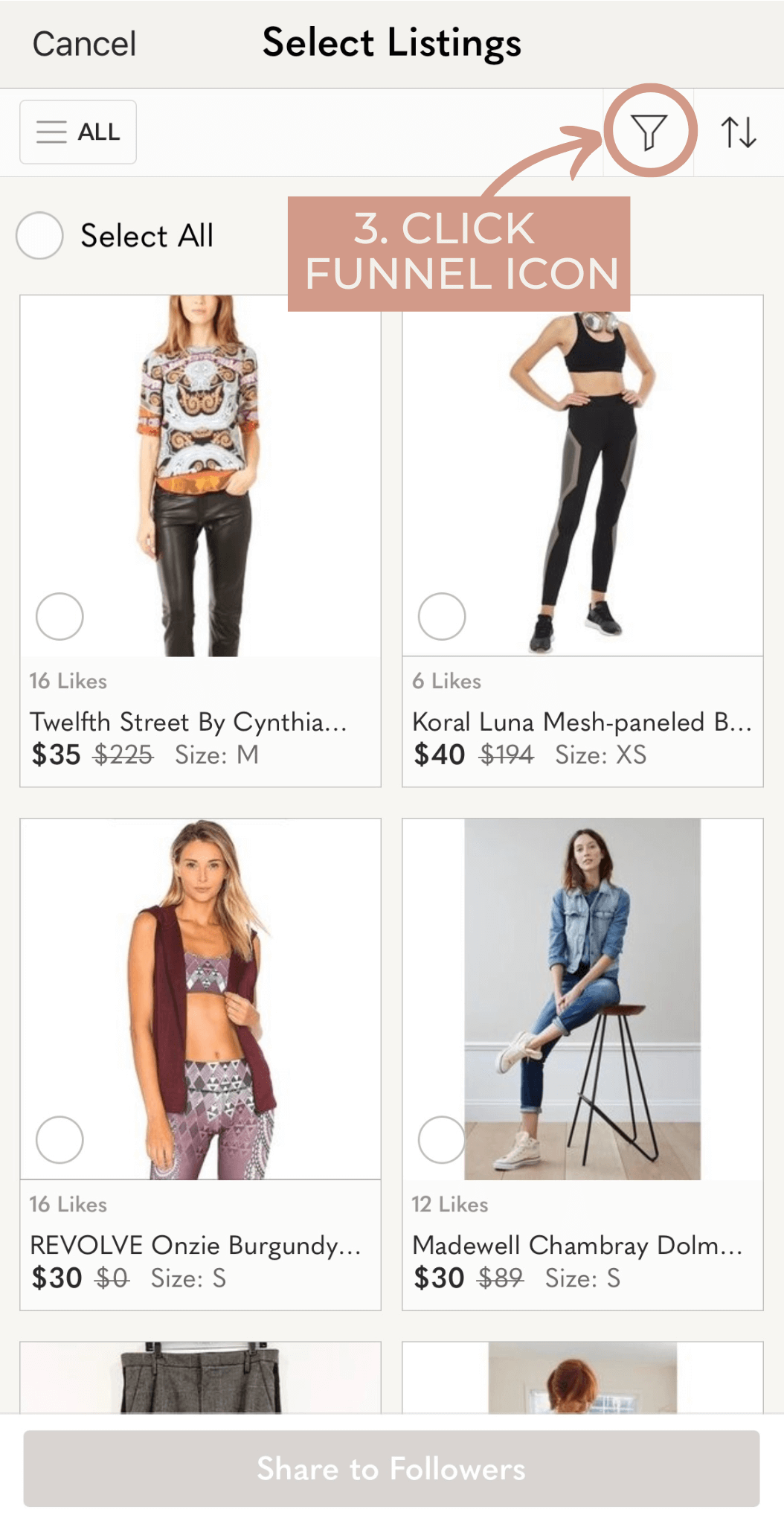The image is a screenshot from a clothing website's listing page. At the top, there's a heading that reads "Select Listings" accompanied by a funnel icon encircled within a pink circle, located just below and to the right of the heading. Below and to the left of this icon, there's an instructional box labeled "3. Click Funnel Icon." The list displays various clothing options, with some visible items being "12th Street by Cynthia," "Cora Luna Mesh Paneled," "Revolve," "Onsi, Burgundy," and "Madewell, Chambray, Dome." The last two listings are partially cut off and not fully readable.